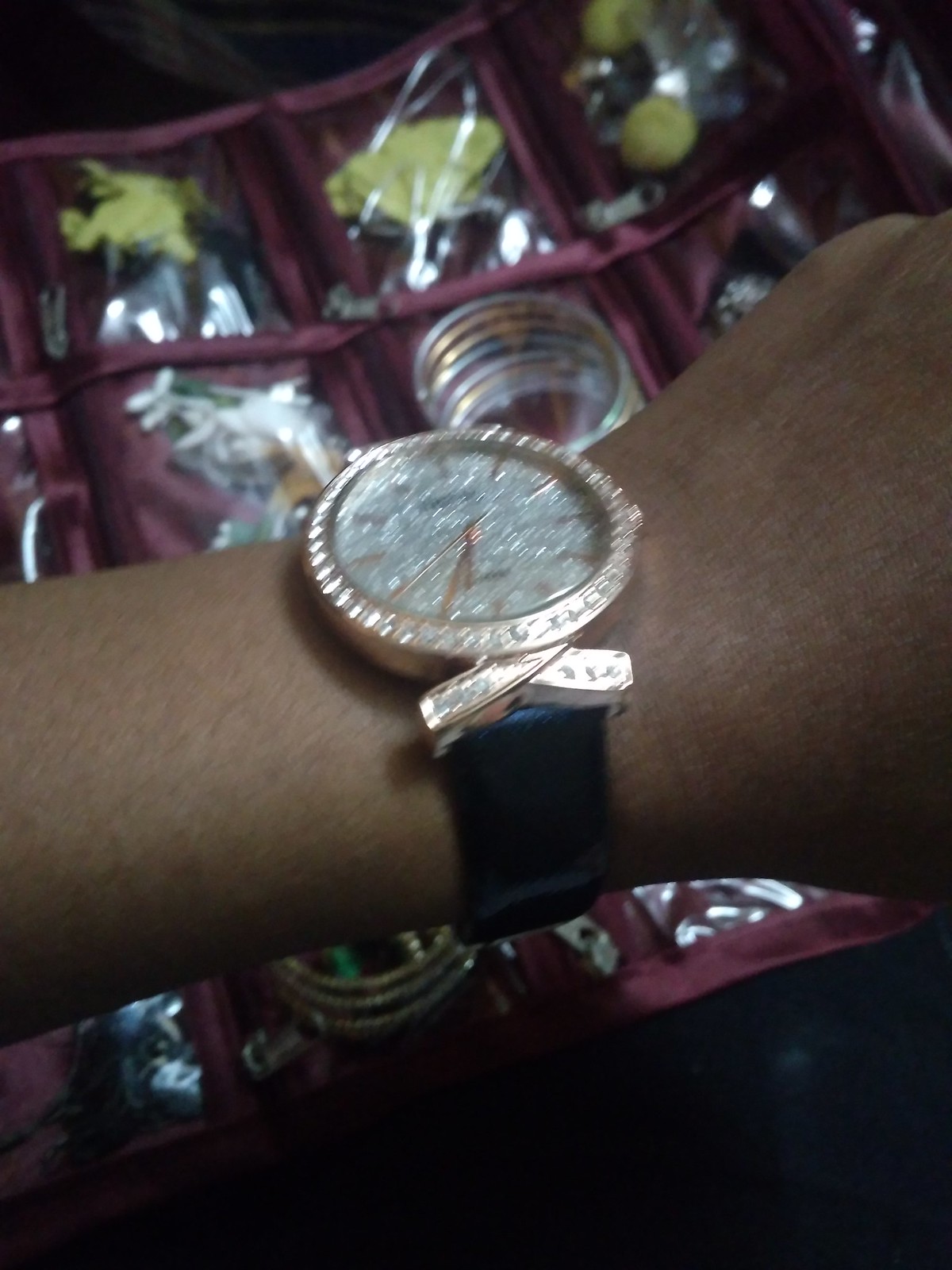The image captures a detailed close-up of a wristwatch modeled on a dark-complexioned wrist. The elegant timepiece features a black leather band and a circular face with a gold border encrusted with diamond-like stones. The watch face itself is adorned with silver glitter, and the gold minute and hour hands stand out against this sparkling background. The watch’s outer rim is embedded with what appears to be Swarovski crystals, giving it an even more luxurious appearance. This intricate design is encased in a reflective material, presumably glass.

In the background, there is a maroon or purple-colored jewelry organizer. This accessory storage unit features multiple zippers and clear plastic sections, providing a glimpse of several items stored within, including various types of jewelry in shades of yellow, black, silver, and gold. The organizer appears to be a practical and stylish solution for keeping jewelry neatly arranged.